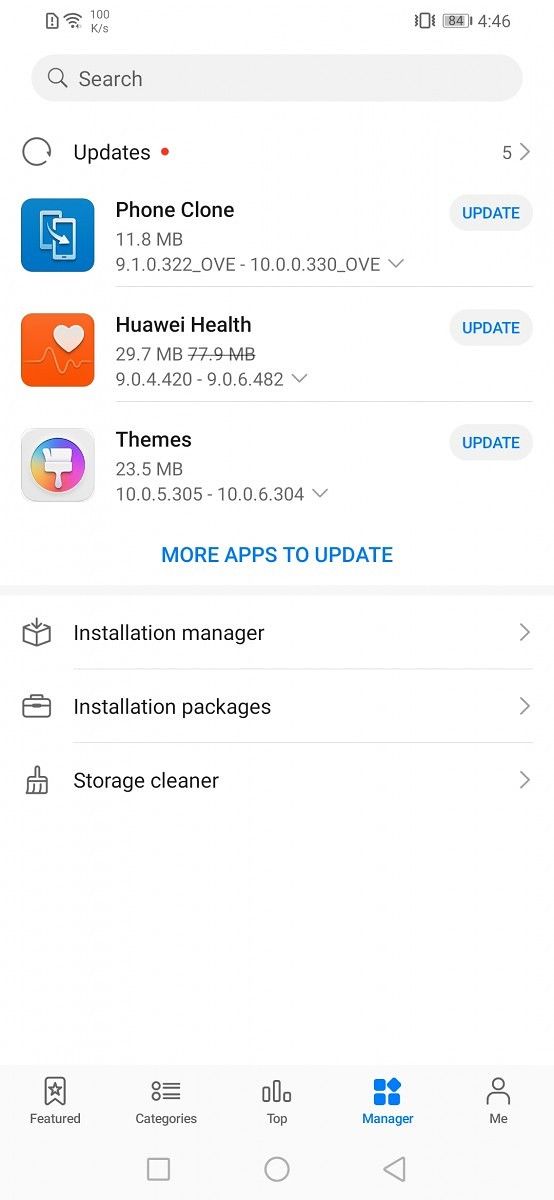In this image, we are looking at a detailed screenshot set against a solid white background. In the upper left corner, the status bar indicates that the Wi-Fi is on, showing a transfer speed of 100 Kbps. In the upper right corner, the battery level is displayed at 84%, and the time is 4:46.

Directly below the status bar, there is a light gray search bar. Beneath it, there's a section titled "Updates (5)" with an arrow pointing to the right. Following this, there is a blue box featuring an image of cell phones, labeled "Phone Clone," with a file size of 11.8 MB. The app version provided is 9.1.0.322 OVE / 10.0.0.330 OVE.

Below "Phone Clone," there's an orange box displaying a heart icon, labeled "WHOE Health," with a size of 29.7 MB. Following this is another app called "Themes," indicated by a white square with a paintbrush over a rainbow background, with a size of 23.5 MB. Each of these three apps has an "Update" button located to their right.

At the bottom of this section, in blue text, are the words "More apps to update."